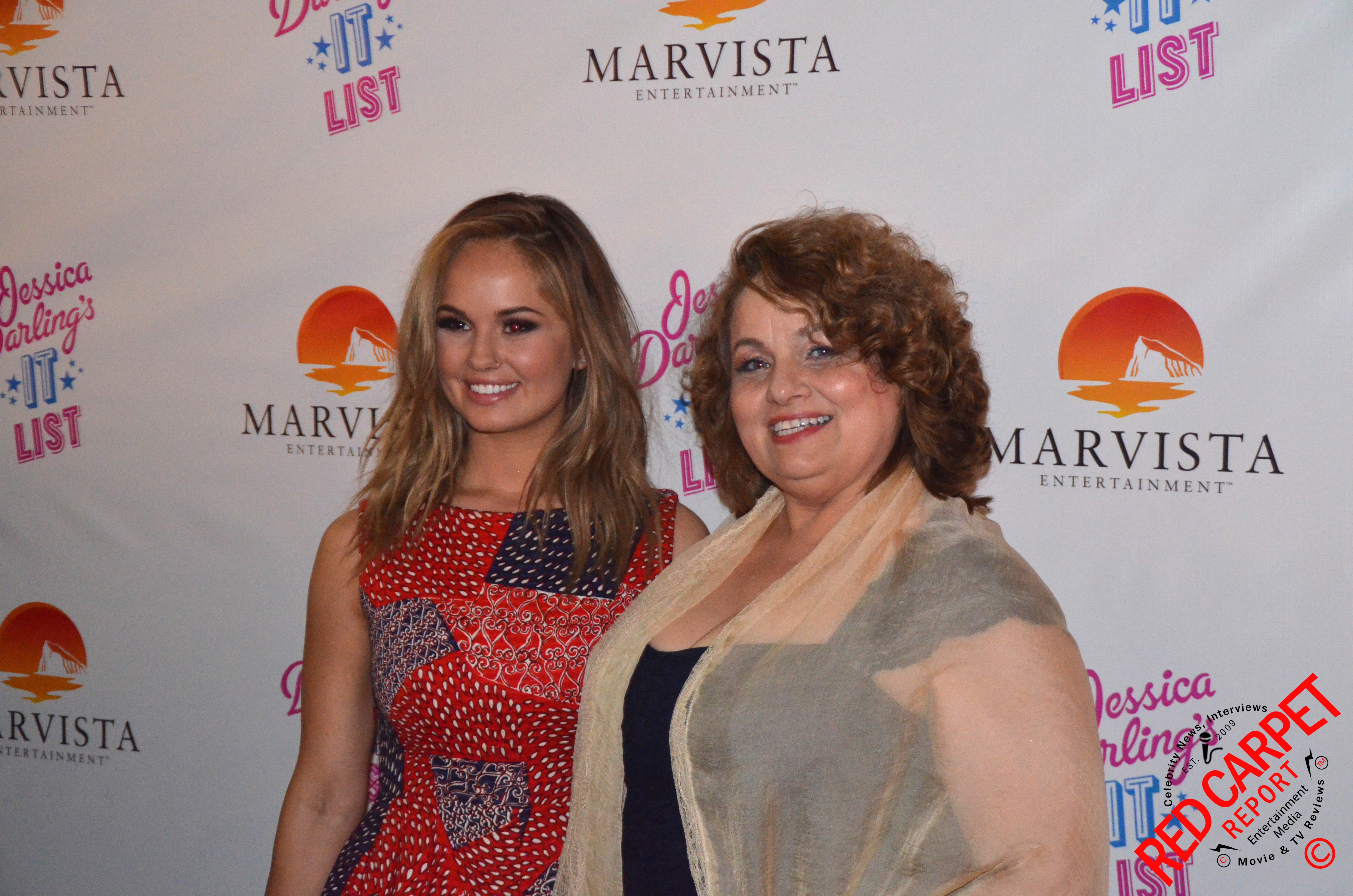In this image, we see two women standing side by side at an event, likely a red carpet meetup, as indicated by the "Red Carpet Report" media logo in the bottom right corner. The backdrop is a white display board with colorful text, including "Mar Vista Entertainment" and "Jessica’s It List."

The woman on the left appears younger, with shoulder-length light brown wavy hair. She is wearing a sleeveless red patterned tank top dress with blue patches. Her makeup is noticeably thick around her eyes, and she is looking straight ahead, smiling warmly.

Next to her is an older, slightly overweight woman with neck-length, messy curly brown hair that has hints of reddish tones, and blue eyes. She is adorned in a black dress with lace cap sleeves, covered by a sheer beige or tan shawl. She has a bright smile, accented with coral lipstick, and is facing the camera directly.

Both women exude a joyful and friendly demeanor against the bright and vibrant event backdrop.